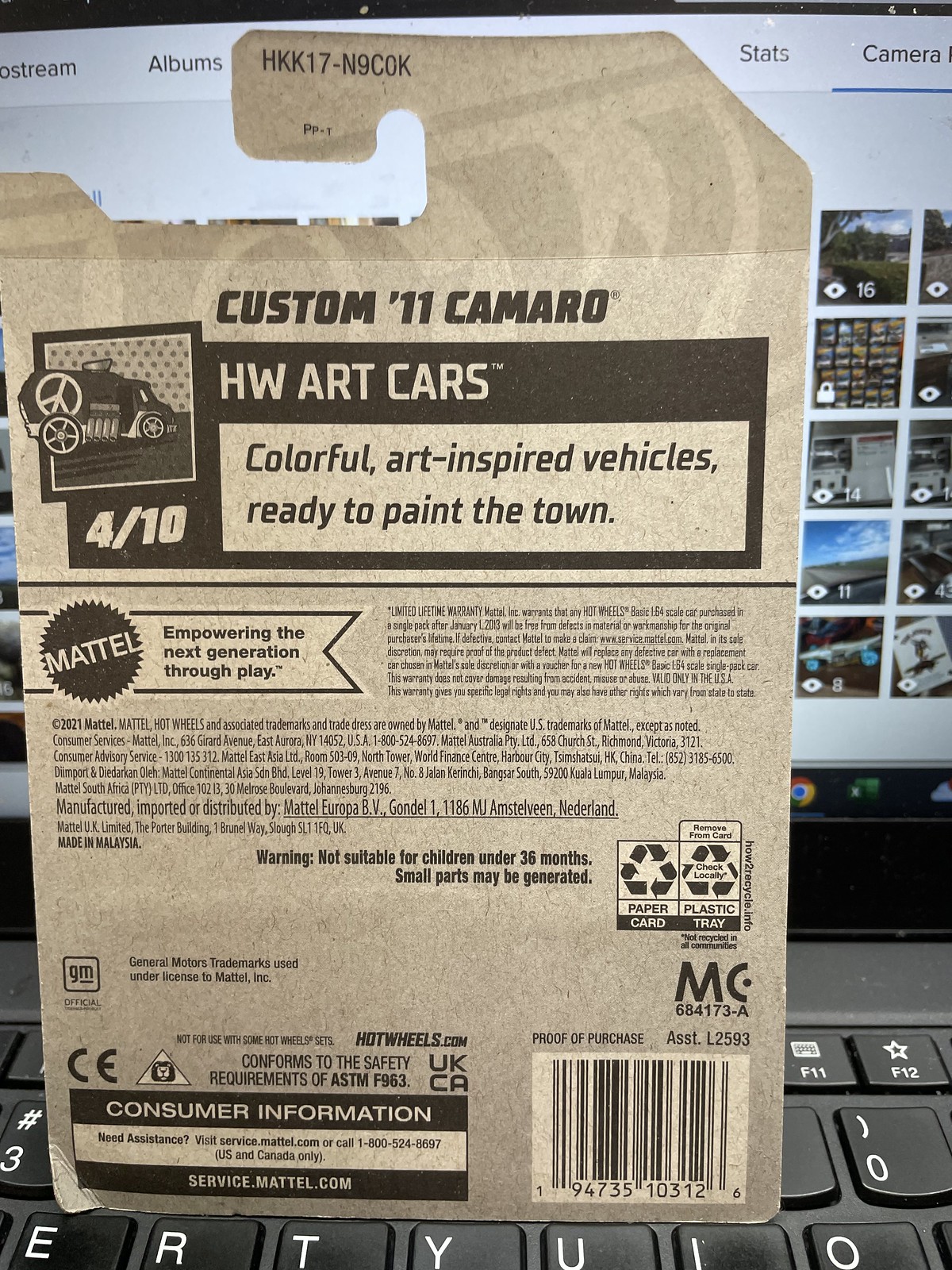The photograph captures a detailed scene with several distinct elements. At the very bottom, a black and white computer keyboard is visible, featuring the keys E, R, T, Y, U, I, N, and O. Standing upright in front of a computer monitor is the backside of a Hot Wheels packaging for a Custom 11 Camaro. The gray, black, and white package has a hook at the top for hanging, likely on a store shelf. 

Prominent text on the packaging includes "Custom 11 Camaro," "HW Art Cars" in a dark box, and "4/10." The slogan "Colorful Art-Inspired Vehicles Ready to Paint the Town" is featured prominently, along with the Mattel logo on the left side, accompanied by the phrase "Empowering the Next Generation through Play." The bottom right of the package contains a barcode, recycling symbols, and very small print.

Behind the Hot Wheels package is a computer monitor displaying numerous small images arranged in a grid with text at the top that reads "Albums," "Stats," and "Camera." The keyboard's presence at the bottom of the image and the numerous images on the computer screen behind it suggest a workspace set up for digital editing or organization.